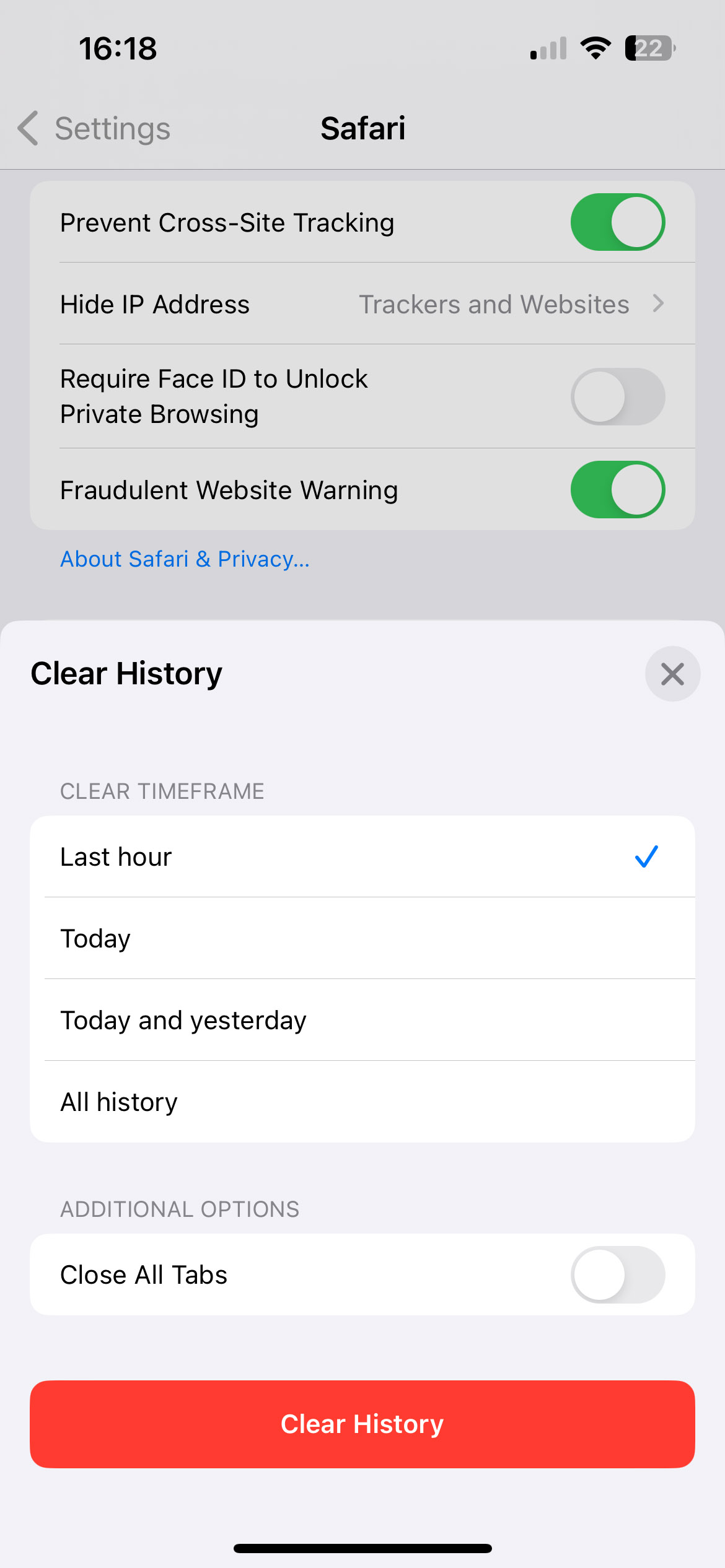This is a detailed screenshot taken from a phone's settings menu, specifically during the time of 16:18 (4:18 PM). The notification bar at the top of the image shows a nearly full Wi-Fi signal, one out of four bars of cellular signal, and a battery level at 22% with the number "22" displayed inside the battery icon.

Beneath the notification bar, there's a back arrow labeled "Settings" on the left side, indicating a navigation option. In the center, the title "Safari" is displayed prominently. The screenshot captures various options under Safari's settings, which include:

1. "Prevent Cross-Site Tracking" - This is toggled on.
2. "Hide IP Address" - Settings for this are partially visible.
3. "Require Face ID to Unlock Private Browsing" - This option is also toggled on.
4. "Fraudulent Website Warning" - This is toggled on as well.

Further down, there are sections for privacy and browsing history:
1. "About Safari & Privacy" - Likely links to more information about Safari's privacy policies.
2. "Clear History" - This section includes an X and a circle on the right-hand side for deletion options.
3. "Clear Time Frame" - Options here include "last hour" (which is selected with a blue checkmark), "today," "today and yesterday," and "all history."

Lastly, there are additional options at the bottom:
1. "Close All Tabs" - This option is toggled off.
2. A red "Clear History" button is located below these settings. 

The overall layout suggests a standard iPhone interface with options precisely related to Safari's privacy and browsing data.